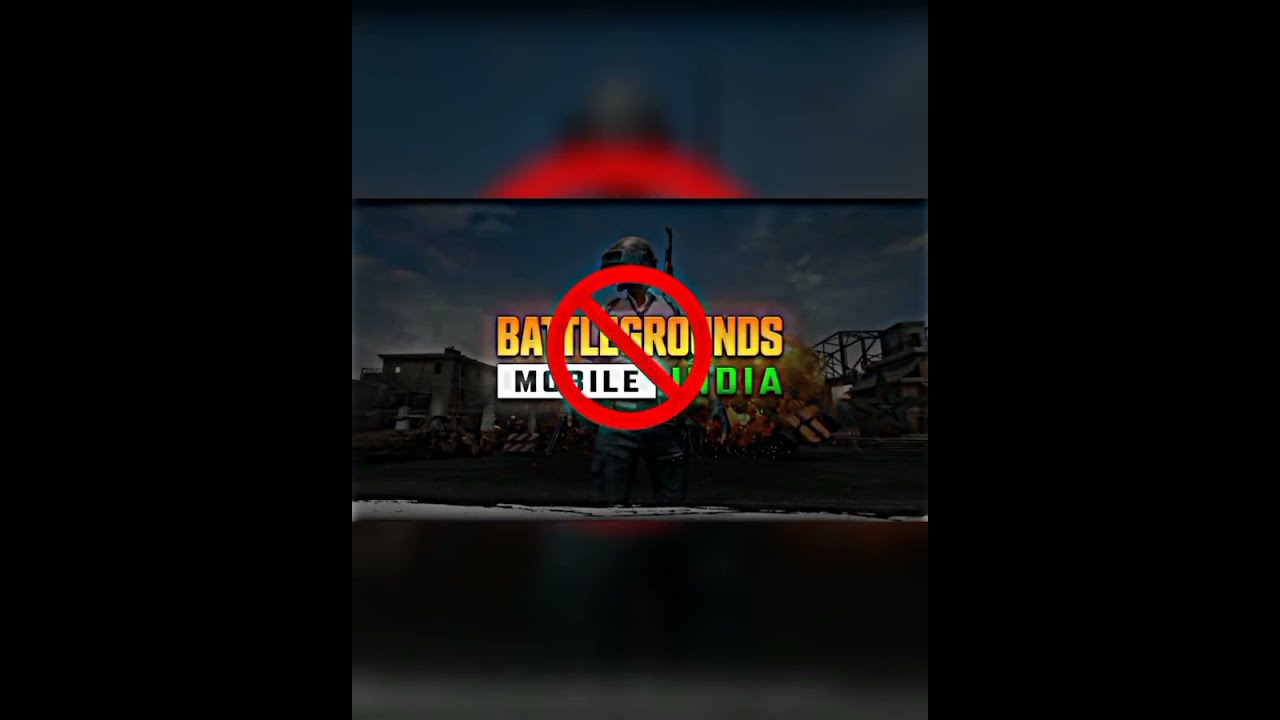The image depicts the logo for the game Battlegrounds Mobile India, set against an apocalyptic backdrop. The background features a dark, cloudy sky with hues of blue and gray, as well as partially visible buildings, piles of debris, and one building to the right that appears to be exploding. In the foreground, a player character is prominently displayed, wearing a white shirt, blue pants, a silver helmet with a strip visor, and a gun strapped to their back. In the center of the image, the game title is written in bold capital letters: "BATTLEGROUNDS" in yellow, "MOBILE" in black within a white box, and "INDIA" in neon green. Overlaying the title is a red circle with a diagonal slash through it, suggesting a prohibited or restricted status. The overall scene is dimly lit, with black bars on each side of the image.